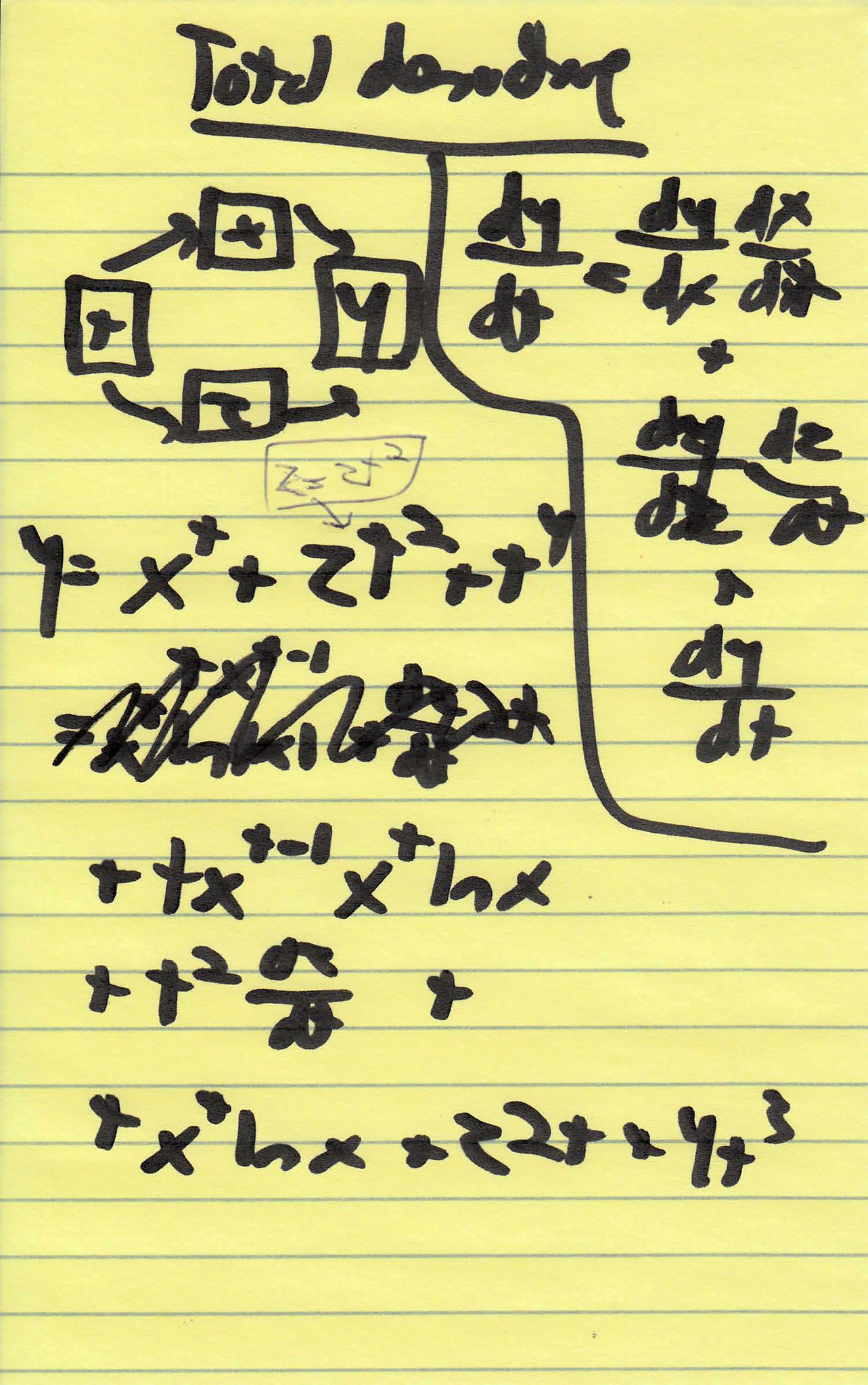A detailed caption for the image could be:

"This image showcases a handwritten mathematical equation on a lined sheet of paper, created using a black marker. At the top of the sheet, a line separates the title from the rest of the content. The main content features an addition problem, with portions of the formula sectioned off for clarity. In the center of the page, blue ink highlights a specific part of the formula that someone is trying to solve. Additionally, a segment of the equation appears to be circular in form, with annotations and workings out written beneath it. A section in the middle of the page has been scribbled out, possibly indicating a correction. At the bottom, the entire formula is meticulously detailed, offering a comprehensive view of the mathematical problem at hand."